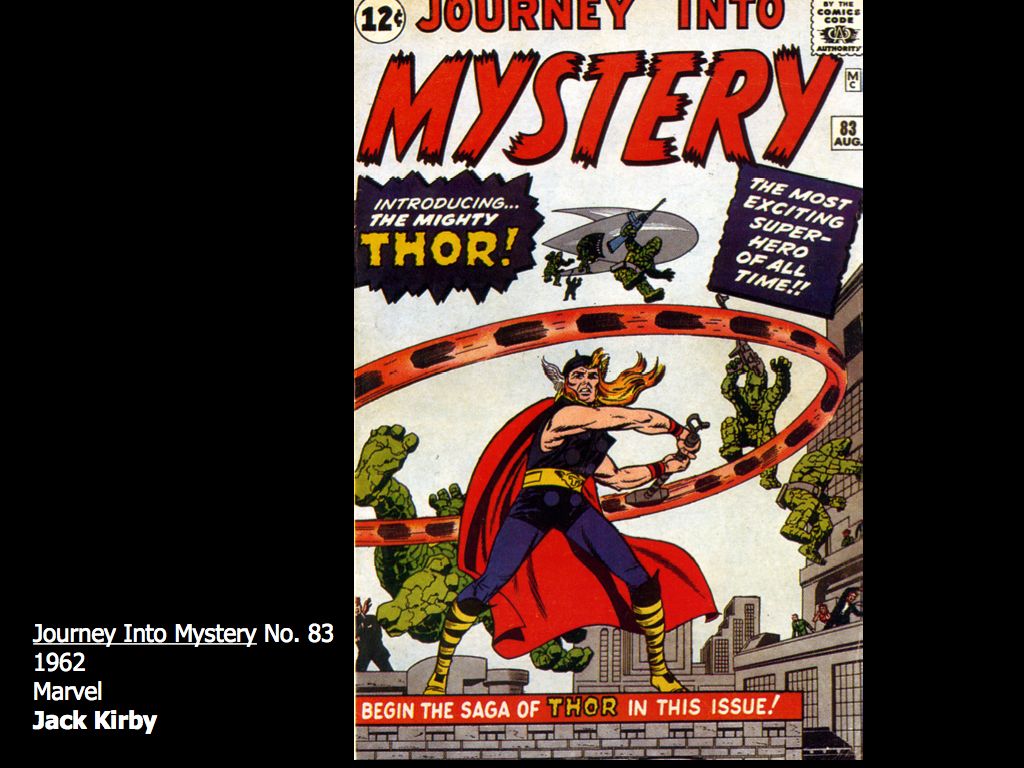This image displays a detailed view of a classic comic book cover set against a plain black background. The comic book cover, a tall vertical rectangle, is positioned just to the right of the image's center. On the black portion of the bottom left of the image, there's white text reading "Journey into Mystery" which is underlined, followed by "number 83, 1962, Marvel, Jack Kirby" not underlined.

The comic cover features a white background with the title "Journey into Mystery" in large, bright red letters at the top. Beneath the title, a purple jagged oval with white text announces "Introducing the Mighty Thor," with "Thor" highlighted in yellow. Prominently showcased is the superhero Thor, who has long blonde hair, a bright red cape, and wears a predominantly purple and yellow outfit. Thor is depicted spinning his silver hammer in a circle, combating green stone creatures emerging from a silver blimp above him.

Further details on the cover include a navy blue box on the left side stating, "Introducing the Mighty Thor," and a red banner at the bottom proclaiming "Begin the saga of Thor in this issue." The comic book initially sold for 12 cents, indicating its vintage status as a valuable collectible from 1962.